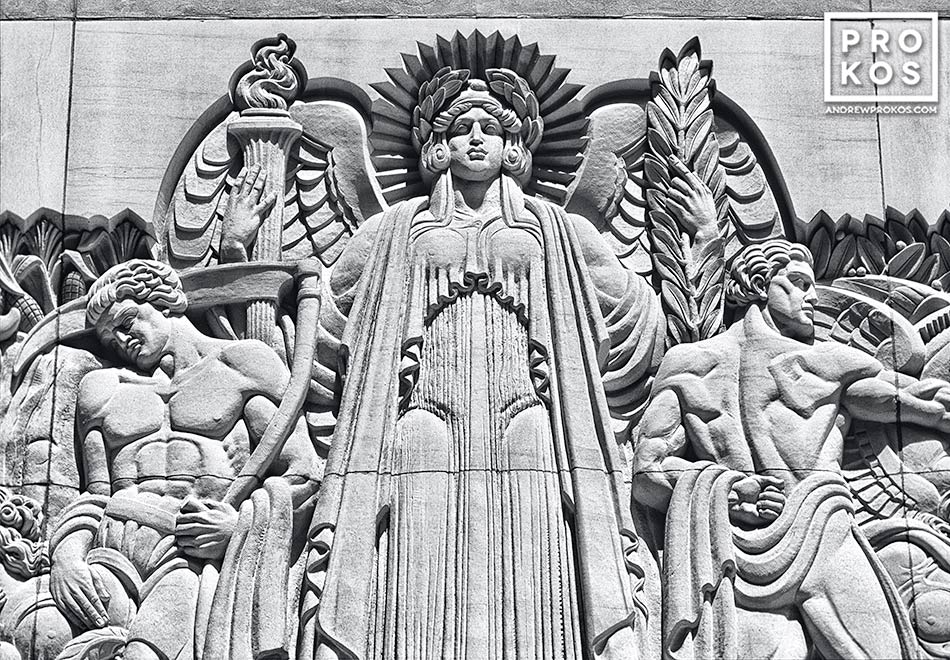The image is a detailed digital photograph of an intricate carving on the side of a building, showcasing a central female figure flanked by two male figures. The sculpture is rendered in shades of white and gray, giving it a timeless, stone-like appearance. The central figure, a woman, is depicted with a crown made of sharp-pointed leaves and angelic wings extending from her back. She wears a flowing robe that outlines her bosom and holds a torch with flames emanating from it. On either side of her, the muscular male figures are shirtless, clad only in loincloths that cover their midsections. The entire scene exudes an air of ancient grandeur and spiritual symbolism. The carving also bears the text "andrewporkrose.com," adding a modern attribution to this classical artwork.